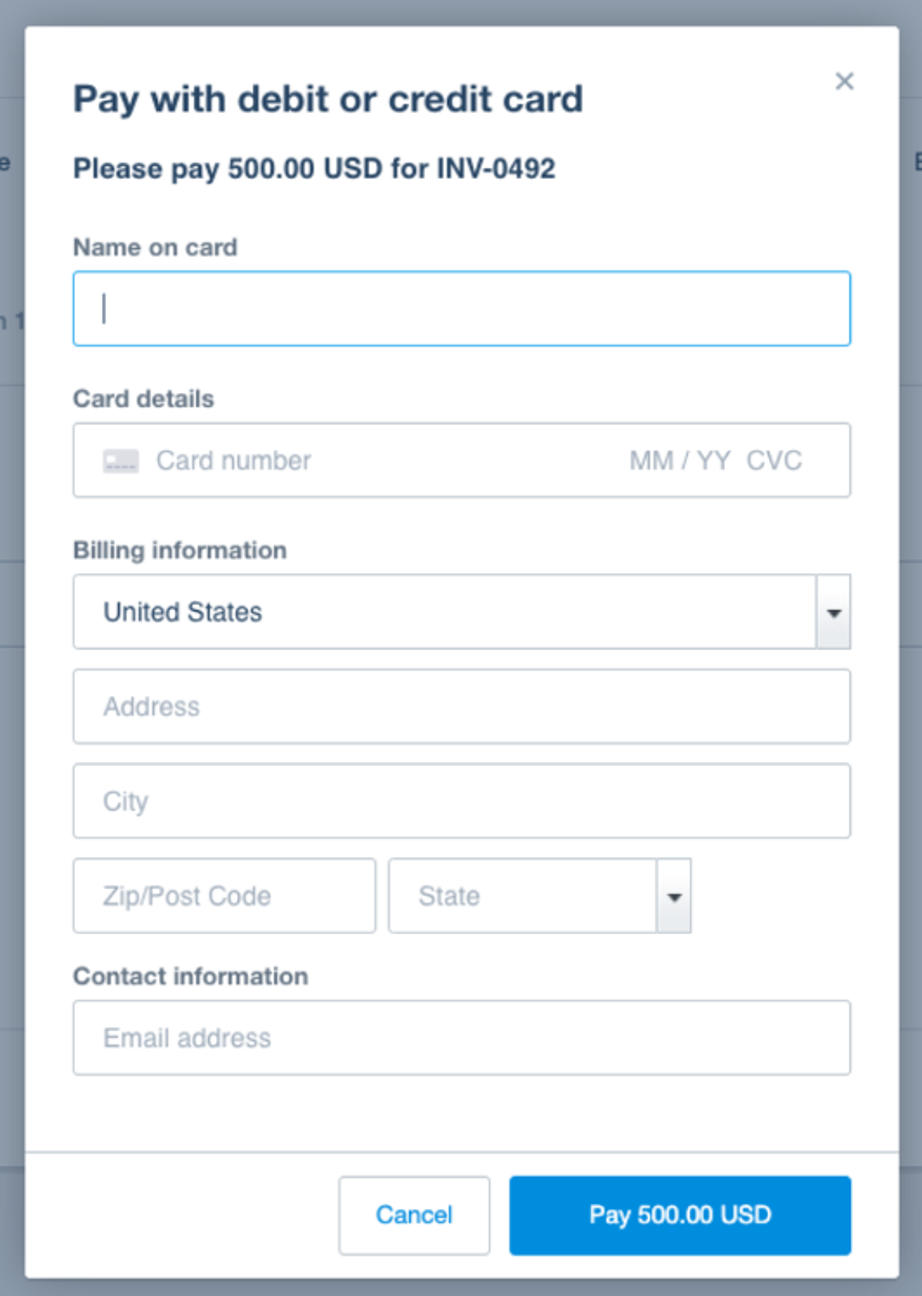Screenshot of a Payment Form Interface

This screenshot captures a vertical rectangular payment form interface from an unknown source, which is outlined with a dark gray border. The interface features the following text and fields:

- **Title:** "Pay with Debit or Credit Card"
- **Payment Request:** "Please pay $500 USD for INV-0492"
- **Card Information Fields:**
  - Name on Card
  - Card Number
  - Expiration Date (MM/YY)
  - CVC

- **Billing Information Fields (with drop-down menus for some):**
  - Country: United States
  - Address
  - City
  - ZIP/Postcode
  - State

- **Contact Information Field:**
  - Email Address

Additional Elements:
- **Action Buttons:** 
  - To the right side, a blue rectangle button labeled "Pay $500 USD"
  - Below the form, a "Cancel" option

This image is purely textual, without any photographic or illustrative elements. There are no people, animals, plants, flags, signs, vehicles, or other visual items depicted. The focus is solely on the information input fields and instructions for completing a $500 USD payment via debit or credit card.